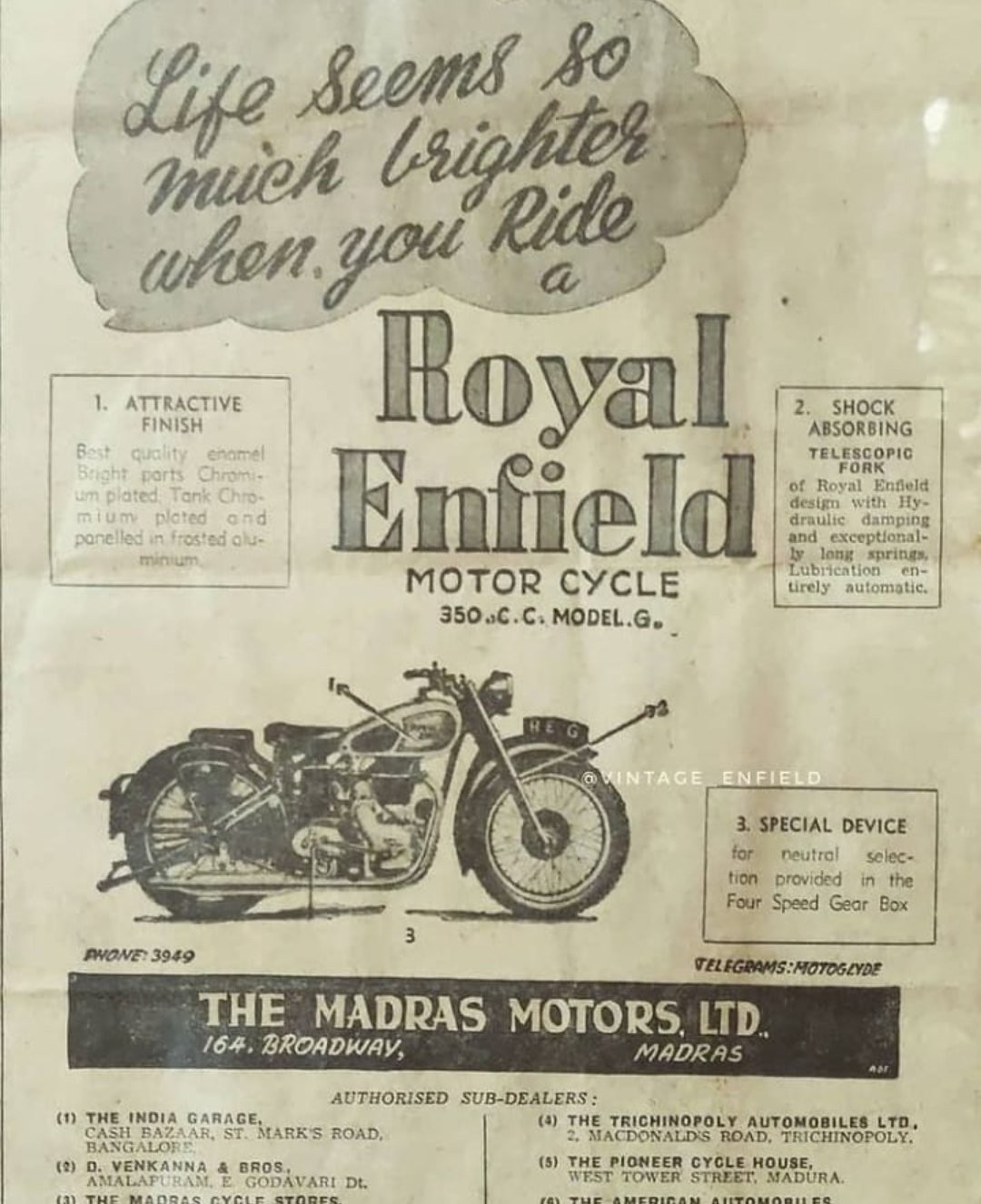This rectangular black-and-white advertisement for the Royal Enfield motorcycle appears to be a page from an old, discolored newspaper or magazine, heavily tinged with yellowish-brown and sporting dirt stains. At the top left, there is a large, light gray cloud or bubble with black cursive text proclaiming, "Life seems so much brighter when you ride." Below this, in gray print, it reads, "Royal Enfield," and further underneath, in black print, it states, "motorcycle 350cc model G." 

Central to the page is a detailed drawing of the Royal Enfield 350cc Model G motorcycle, facing left to right, without a windshield. The motorcycle illustration is accentuated by arrows pointing to specific parts, although the labels are too small to decipher clearly. Surrounding the motorcycle are three boxes: one on the left labeled "1. Attractive Finish," one on the right labeled "2. Shock-absorbing telescopic fork," and beneath it, labeled "3. Special Device."

Directly below the motorcycle, there is a small notation: "Phone 3949" on the left. A black banner runs across the bottom of the page, with white print stating, "The Madras Motors LTD, 164 Broadway, Madras." Smaller, hard-to-read text runs under this banner, which is split into sections listing authorized sub-dealers. These include:
1. India Garage
2. D. Van Kana & Bros.
3. Madras Cycle Stores
4. Tricanopoly Automobiles LTD
5. Pioneer Cycle House
6. American Automobiles.

Above the list of sub-dealers, there are instructions for telegrams addressed to "Motoglide."

The advertisement encapsulates the vintage charm and technical allure of the Royal Enfield motorcycle, highlighting its attractive finish and advanced shock-absorbing features while providing essential contact information and authorized dealership details.